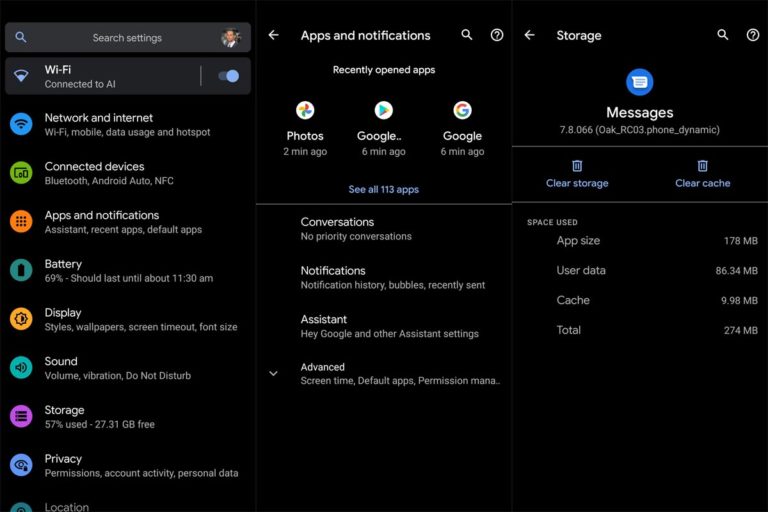The image displays a computer screen with a black background, showcasing what appears to be a control panel. At the top of the screen, there are options for "Search settings." 

On the left-hand side, centrally located, is a section labeled "Apps and notifications." To the right of that, there is a section labeled "Storage." Further to the far right, a small magnifying glass icon represents a search feature, and next to it, a small circle with a question mark signifies help.

On the left-hand side of the screen are several options listed vertically: 
- Wi-Fi
- Network & internet
- Connected devices
- Apps & notifications
- Battery
- Display
- Sound
- Storage
- Privacy
- Location

In the central part of the screen, there are three circular icons: 
- The leftmost icon represents "Photos."
- The center icon appears to be related to Google Play, identified by a right arrow within the App icon.
- The rightmost icon is a large 'G' within a circle, representing Google.

Below these icons, under the section titled "Recently opened apps," it reads "See all 113 apps." This section also includes categories such as "Conversations," "Notifications," "Assistant," and "Advanced."

On the rightmost side of the screen, there is a blue circular app icon featuring a small white page, which is labeled "Messages." Beneath this label, there are two options:
- The left icon is a small garbage can labeled "Clear storage."
- The right icon is another small garbage can labeled "Clear cache."

Under "Space used," the details provided are:
- App size
- User data
- Cache
- Total